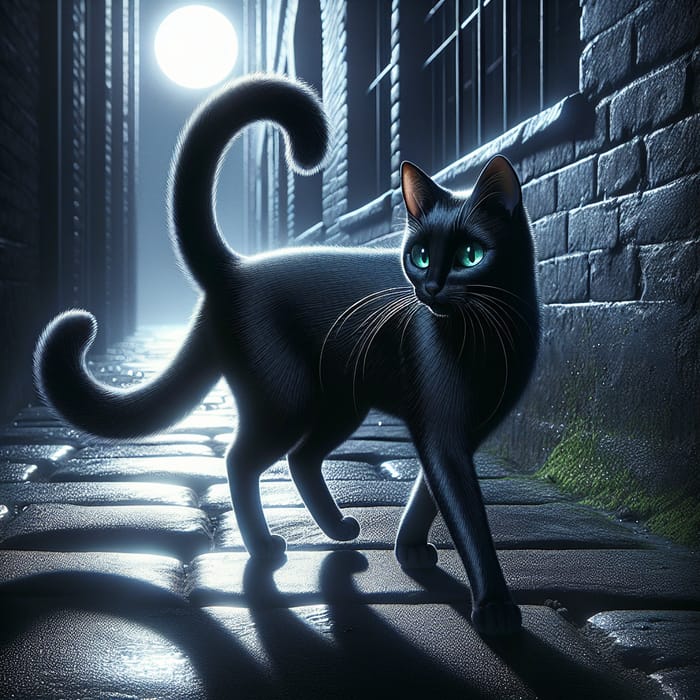This square image appears to be an AI-generated artwork, featuring a black cat with two tails standing in a cobblestone alleyway at night. Illuminated by a full moon shining on the scene, the cat has bright green eyes and very long whiskers that stand out against its dark fur. One of its tails curls up above its back while the other curves lower to the ground, together forming a sideways 'S' shape. The alley is nestled between two buildings: a dark-painted concrete block on the left and a brick or stone structure on the right, which has bars on an upper window and a patch of grass at its base. The night setting adds a mysterious ambiance, with the rough, textured cobblestones and the generally black and gray tones of the image enhancing the eerie atmosphere.